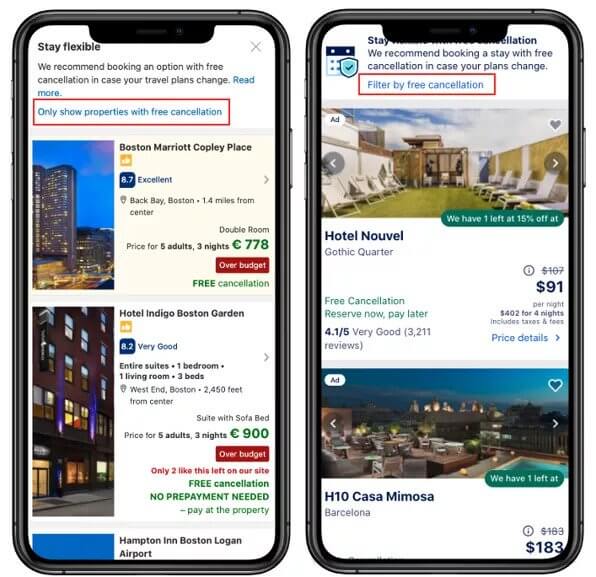The image consists of two side-by-side phone screenshots, both showing the same travel booking app with identical dimensions and shape, highlighting the outlines of the phones themselves. Each screenshot displays different aspects of hotel searches. 

### Left Screenshot:
- **Background:** White
- **Text Color:** Dark Blue
- **Highlighted Message:** "Stay flexible. We recommend booking an option with free cancellation in case your travel plans change. Read more."
- **Highlighted Option:** "Only show properties with free cancellation" outlined in red, potentially selected.
- **Currency Display:** Prices are shown in euros (€).
- **Listings:**
  1. **Boston Marriott Copley Place** - Price: €778.
     - Accompanied by a thumbnail photo.
  2. **Hotel Indigo Boston Garden** - Price: €900.
     - Accompanied by a thumbnail photo.

### Right Screenshot:
- **Background and Text Layout:** Identical to the left screenshot but displaying prices in US dollars ($).
- **Listings:**
  1. **Hotel Nouvelle Gothic Quarter** - Price: $91.
     - Accompanied by a photo showing a bunch of pool chairs.
  2. **Casa Mimosa Barcelona** - Price: $183.
     - Accompanied by an illustrative photo.

The descriptive captions provide a clear comparison between hotel listings in euros and US dollars, highlighting various properties and their respective prices.